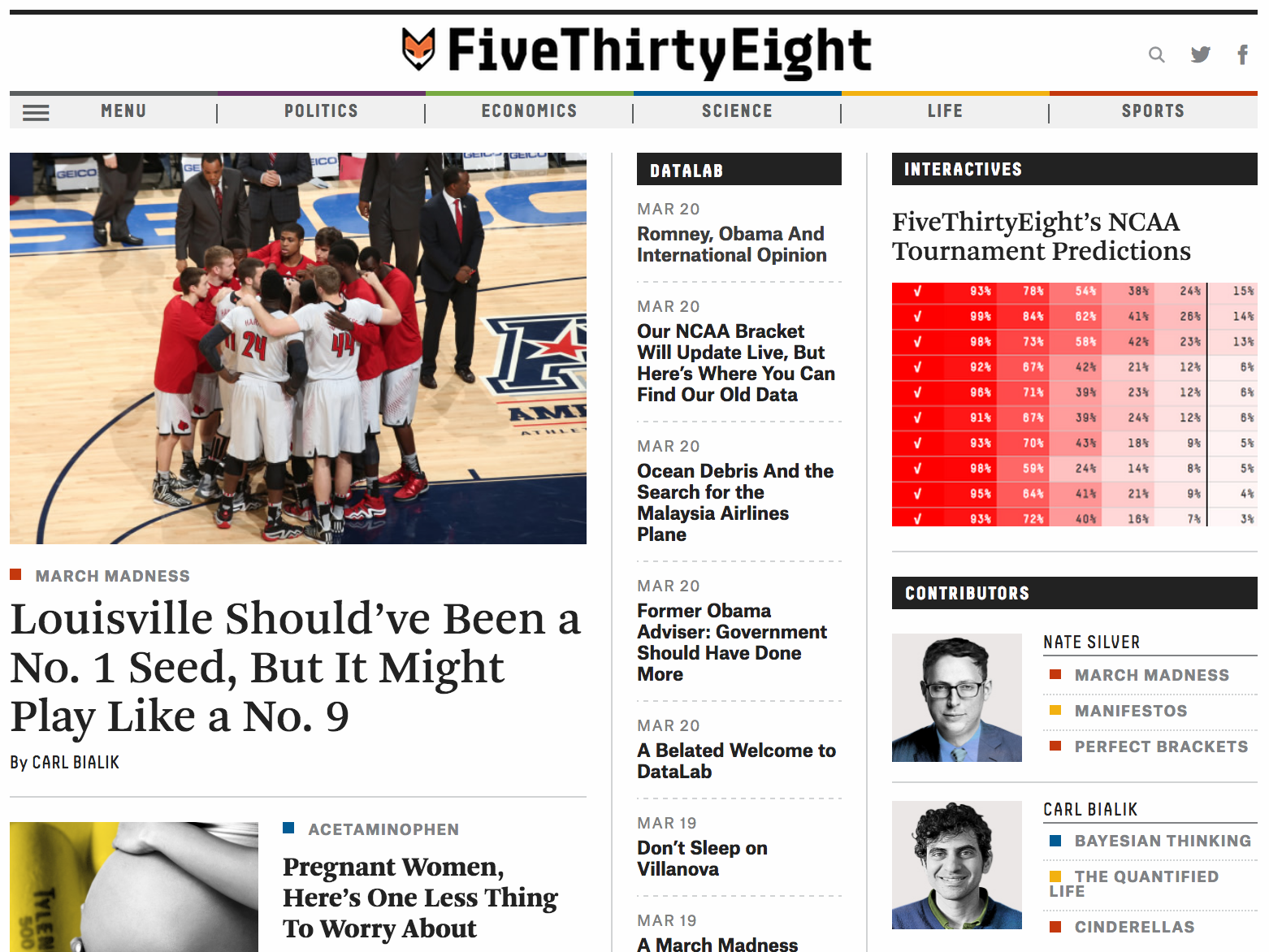This is an image of a webpage showing a detailed layout of its interface. At the top, a horizontal black line spans the entire width from left to right. Below this, prominently in the center, is an intricate artwork of a fox, with colors black, orange, and white. To the right of the fox, the webpage displays the number "538." Adjacent to this number is a row of icons: a magnifying glass symbolizing the search function, a Twitter icon, and a Facebook icon, arranged sequentially from left to right.

Below these elements, a navigation bar runs horizontally, featuring several tabs labeled in an orderly fashion: Menu, Politics, Economics, Science, Life, and Sports.

In the lower section of the webpage, positioned on the left side, there is an image depicting a group of basketball players on a court. Several players are wearing coordinated white jerseys and shorts, while some players in the background are dressed in red tops. Additionally, a few individuals wearing black suits can be seen in the background, behind the players.